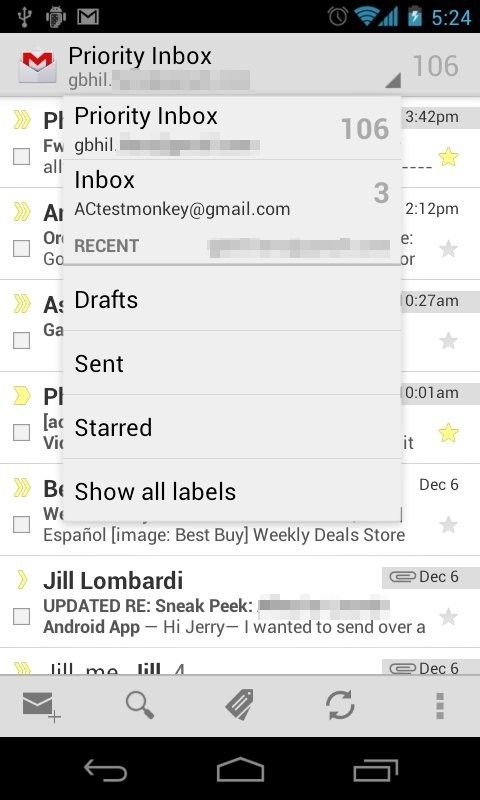A screenshot from a smartphone display shows the Gmail app open to the Priority Inbox. At the top middle of the screen, a smaller overlay box labeled "Priority Inbox" is visible. It includes text with the words "G-B-H-I-L," "Inbox," and the email address "actestmonkey@gmail.com." Some information in this smaller box is blurred out for privacy, specifically near the words "recent" and the email address area. Below this, a faint gray line separates other options such as "Drafts," "Sent," "Starred," and "Show All Labels." In the background of the screenshot, an email from Jill Lombardi is partially visible with subject lines and snippets that read: "Updated, RE sneak peek, Android app. Hi, Jerry. I wanted to send over a..." which is cut off, indicating a partially visible list of inbox emails.